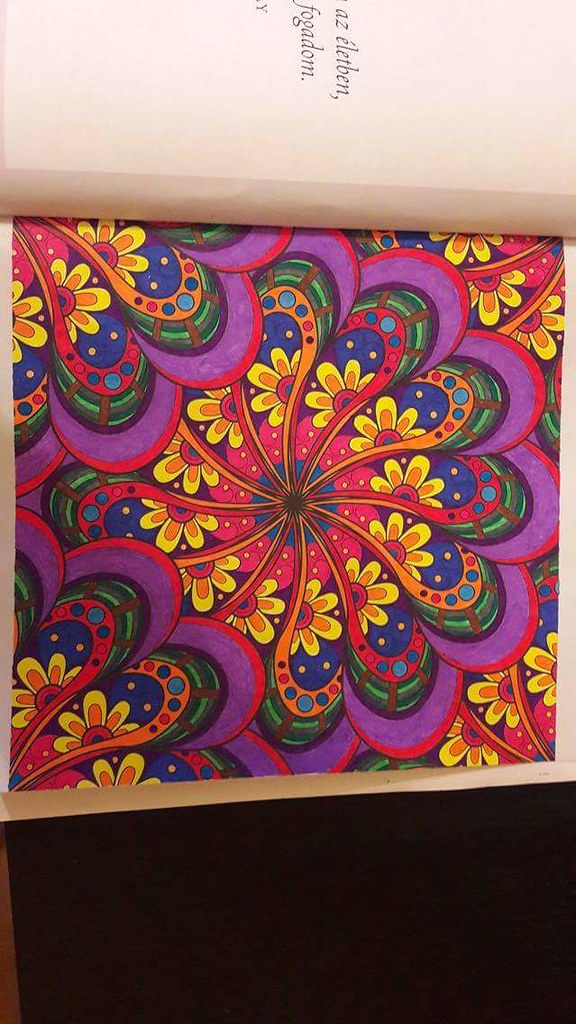This photograph features a vibrant piece of artwork displayed on a card. The bottom quarter of the image is black, providing a striking contrast to the colorful composition above. 

At the center of the artwork is a brown circle surrounded by steel blue triangles, forming a larger circle around it. Emerging from this central design are red, orange, and yellow lines that curve gracefully, resembling question marks, all emanating from the core.

Encircling the blue center is a ring of red adorned with yellow dots. Outside this is a circle of yellow daisies, adding a floral touch. Further out, a half circle of blue with a beige dot in it and a half circle of red or orange with green and red dots are presented. The outermost edge of the artwork is bordered by a red ring with a purple interior.

This intricate design evokes a sense of whimsy, reminiscent of a child's drawing of a daisy, with additional daisies embellishing each corner of the artwork.